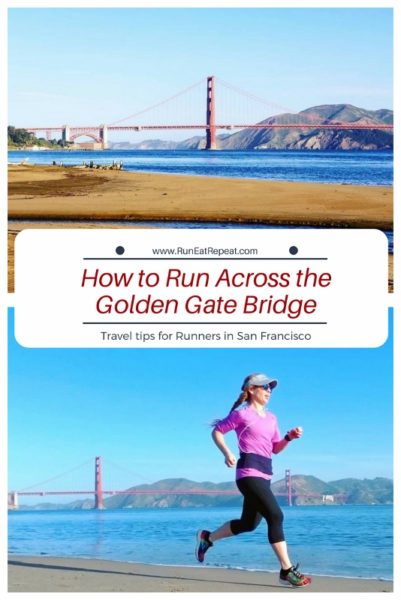This image appears to be a guide titled "How to Run Across the Golden Gate Bridge" with travel tips specifically for runners in San Francisco. The guide prominently features the URL www.runeatrepeat.com written in small black print at the top and travel tips for runners in San Francisco at the bottom.

The top part of the image showcases a picturesque view of the Golden Gate Bridge against a bright blue sky, deep blue waters, and a sandy beach with brown sand. Additionally, there are some trees and shrubs off to the side, and a beach scene indicating a pop-up setup, possibly with people and chairs.

Beneath the main title in large red letters, there's a second image depicting a female runner along the water's edge with the iconic Golden Gate Bridge in the background. She is dressed in black capri pants, a hot pink shirt, and rainbow-colored running shoes. She also wears a gray visor, sunglasses, and has her brown hair styled in a braid. A wire, likely for earphones, runs from her waist to her ears, suggesting she is listening to music as she runs.